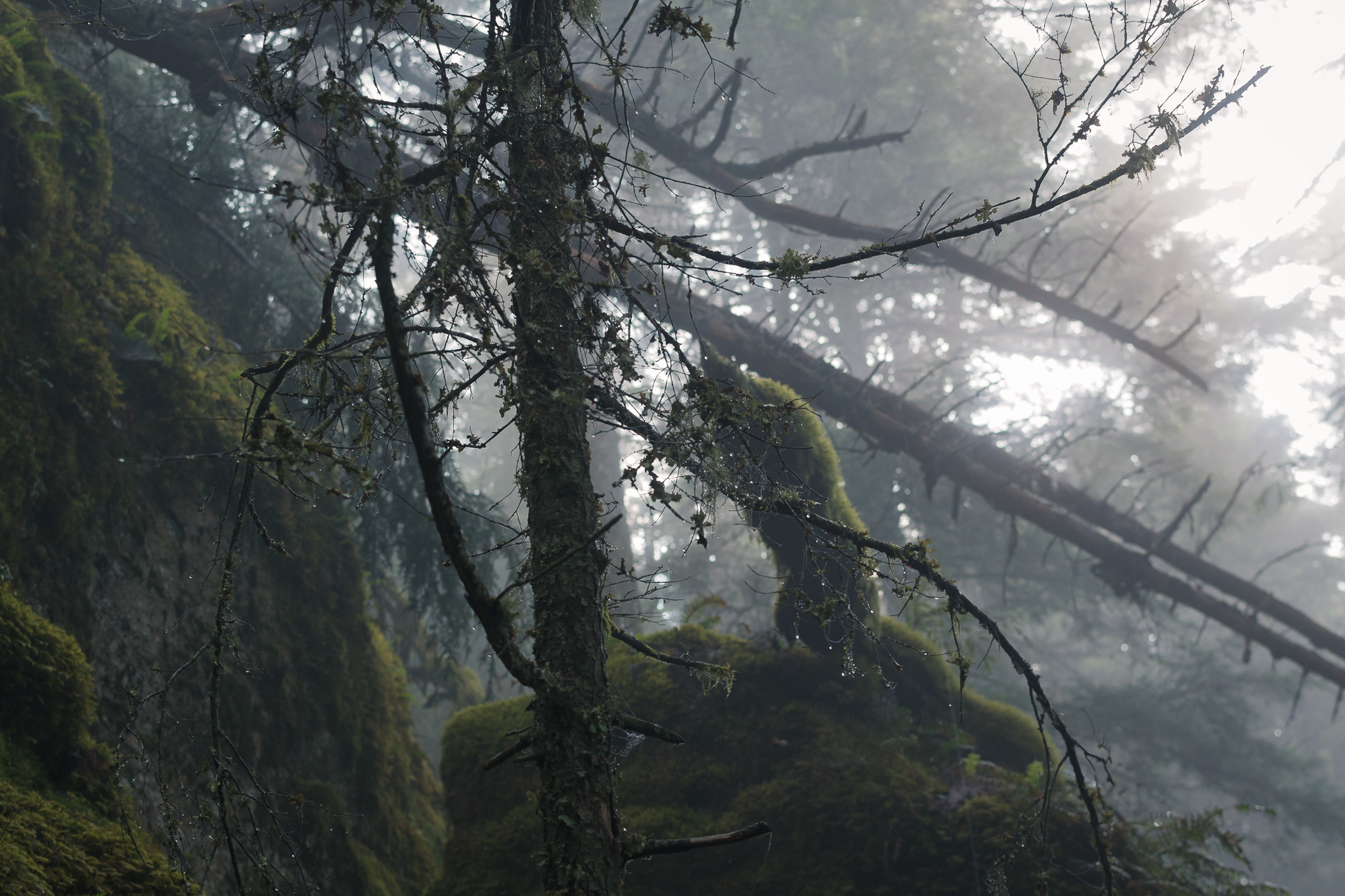A photograph captured in a dense forest reveals a tranquil post-rain scene. Centered in the frame are several dead trees, devoid of leaves, with bare branches reaching out like skeletal fingers. Among these fallen giants, a particular pine tree, now just a network of branches, stands out. The forest floor and the scattered rocks are carpeted with lush, green, and fluffy moss, glistening with tiny dew droplets, hinting at recent rainfall. The scene is predominantly shaded, contributing to a damp atmosphere, save for a bright shaft of sunlight streaming in from the upper-right corner, casting a gentle glow on the mist-kissed elements. The left side of the image remains in shadow, enhancing the contrast between light and dark. In the background, standing in serene contrast to the deceased trees, are tall and robust trees still adorned with their vibrant leaves, adding depth and life to the composition. The photograph captures the serene beauty and quiet aftermath of nature’s gentle shower.